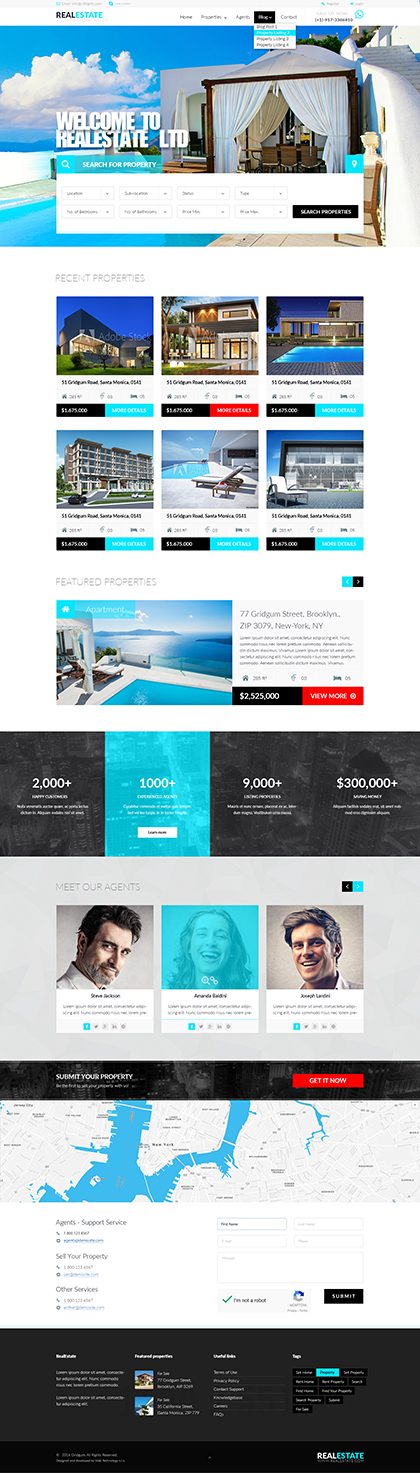The webpage opens with a header displaying various photographs of buildings. At the top, there is an image of gray buildings draped with white coverings. Superimposed on this image in white text is a welcoming message: "Welcome to Real Estate, LTD."

Below the heading, a series of photographs showcase diverse buildings: one gray, one blue, one white, one tan, and another white. Each photograph is accompanied by a descriptive bezel. The first bezel features a black square with "2000" in white text. Following that, a cyan blue square displays "1000." Another bezel reads "9000," and yet another states "300,000."

In the gray section, images of individuals are highlighted. One photograph shows a light-skinned, middle-aged man with a gray beard, black hair, and a white shirt. Adjacent to this, within a cyan blue square, a woman with brown hair is portrayed. On the right side of this section, another photograph depicts a short, light-skinned man with brown hair.

Towards the bottom of the webpage, a map is displayed alongside a substantial amount of text. The text is illegible due to the distant screenshot, but it appears in white against a dark gray bezel. At the very bottom, the words "real" in white and "estate" in cyan blue are prominently shown, framed by a dark gray background. Additionally, the top portion of the page features the words "real" in black and "state" in blue, set against a dark gray bezel.